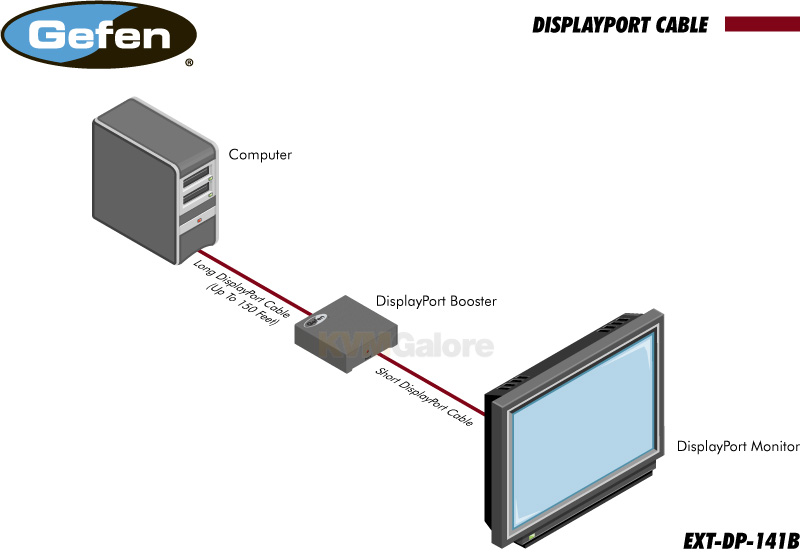The image depicts a detailed diagram for setting up a Geffen computer system and its DisplayPort components. The background is white, and in the upper left corner, there's an egg-shaped oval logo for Geffen, spelled "G-E-F-F-E-N" in mixed-case white letters set against a blue and black split background with a squiggly line in the middle. The diagram illustrates a sequence starting with a computer on the left, followed by a long DisplayPort cable that can extend up to 150 feet, connected to a DisplayPort booster. Another shorter DisplayPort cable extends from the booster to a DisplayPort monitor, which is also labeled as a TV. The serial number EXT-DP-141B is noted in black fonts, providing specific identification for this DisplayPort unit.